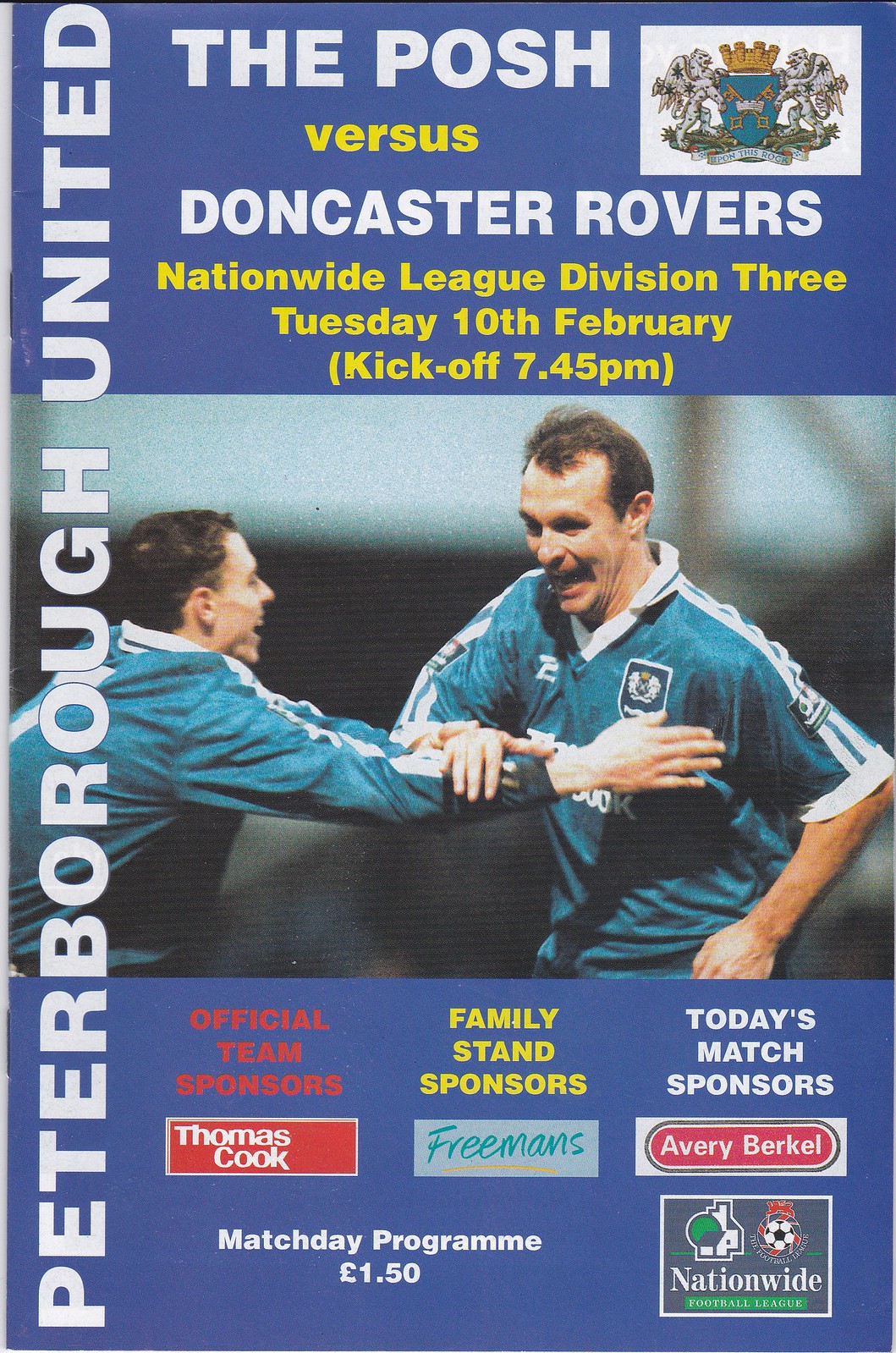This image depicts an old Match Day Program for a UK football match between Peterborough United, known as "The Posh," and Doncaster Rovers in the Nationwide League Division III. The event is scheduled for Tuesday, 10th February, with a kickoff at 7.45 PM. The program features a central photograph of two jubilant soccer players wearing green jerseys, one in short sleeves and the other in long sleeves, celebrating. Above and below the image, a blue background hosts white text detailing the event information. The top section promotes the match details, while the bottom lists the official team sponsors: Thomas Cook, Freemans as the family stand sponsor, and Avery Burkle as today's match sponsor. The program is priced at £1.50. Additionally, there are various symbols, including a crest in the upper right corner with a crown and winged creatures, and a "Nationwide" logo in the lower right corner.